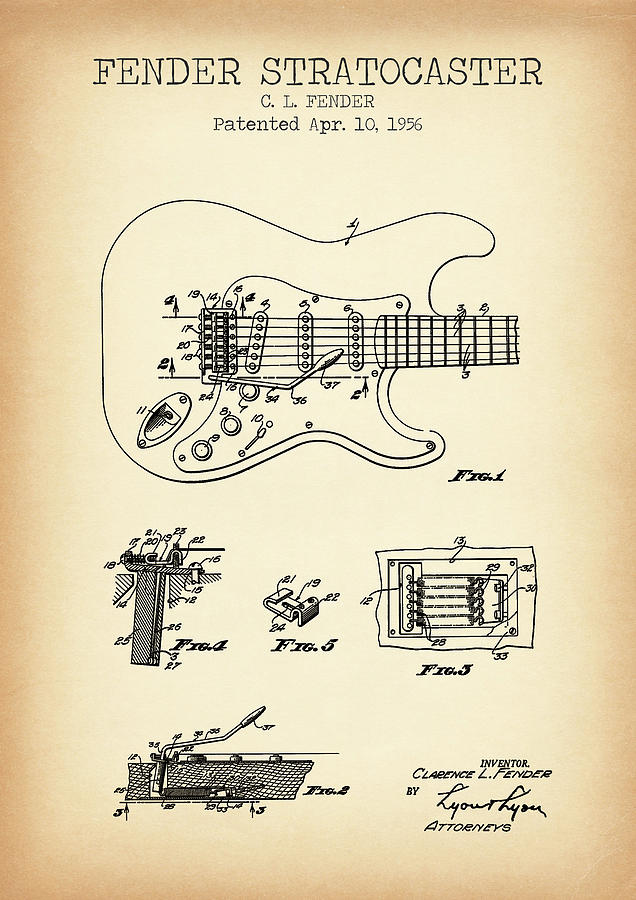This detailed line art diagram of a Fender Stratocaster guitar appears on a pale peachy-salmon background, resembling a piece of parchment. The top of the image reads "Fender Stratocaster, C.L. Fender, Patented April 10, 1956," in a black typewriter-like font. The illustration serves as a patent document showcasing various intricate parts of the guitar. 

The primary drawing, labeled as Figure 1, depicts the fully assembled front view of the guitar. It includes labels pointing to different components such as the frets, pickups, knobs, and input jack. Surrounding this main illustration are smaller, detailed drawings labeled Figures 2 through 5. Figure 2 focuses on the headstock, where the strings are connected. Figure 3 seems to illustrate a metal bracket, while Figure 5 shows the bottom section of the guitar where the strings anchor. Figure 4 appears to detail part of the wiring or electronics inside the guitar.

The document's bottom right corner notes "Inventor Clarence L. Fender by," followed by an illegible handwritten name and the word "Attorneys." This visually rich and detailed layout likely served as the original patent filing for the 1956 Fender Stratocaster guitar.